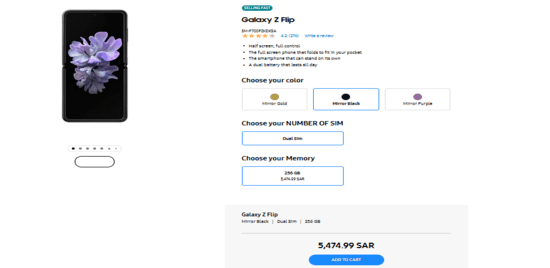The image is a horizontally rectangular screenshot from a product listing for a Galaxy Z Flip cell phone. On the left side of the frame, there is an image of the phone in a portrait position. The phone has an all-black design, accentuated by a bright purple flower displayed in the center of its screen. 

On the right side of the frame, the product details are shown. At the top, "Galaxy Z Flip" is prominently mentioned, accompanied by a four-star rating. Although the text beneath the rating is too small to decipher, it's followed by a section to "choose your color," featuring three horizontal color options, with the black color selected. Below that, there are sections for selecting the "number of SIM" and "memory," each accompanied by a dropdown box for making the selections, though the specific details are unreadable due to the small print.

At the bottom of the listing, the total price of 5,474.99 SAR is displayed, alongside a prominent "add to cart" button.